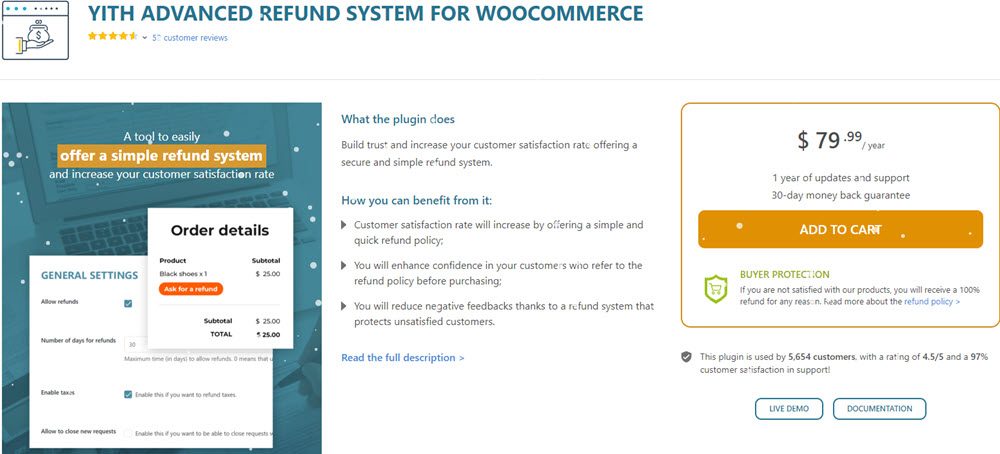This image features a promotional graphic for the "YITH Advanced Refund System for WooCommerce" plugin. The central theme of the image is a comprehensive refund system designed to enhance customer satisfaction. The title "YITH Advanced Refund System for WooCommerce" is prominently displayed, accompanied by a logo depicting a hand holding a bag of money, symbolizing financial transactions.

Set against a green background, the phrase "Refund System" appears in striking orange text to draw attention. Directly below, a tagline in smaller white text emphasizes the benefit: "Increase your customer satisfaction rate."

Toward the left side of the image, a gray box details the simplicity and utility of the tool, with the mention that the system offers easy-to-read features for streamlined refunds.

In the center, a white pop-up box labeled "Order Details" includes an orange oval button for navigation. Behind this, another box highlights "General Settings," indicating where users can configure the plugin. Supplementing this, blue headers with black text underneath explain the functionality and benefits of the plugin. There is also a clickable link to "Read the full description."

On the right, bordered by an orange outline, the pricing information states "$79.99 per year," which includes one year of updates and support with a 30-day money-back guarantee. An orange button offers the option to "Add to Cart." 

Additionally, a green outline highlights a "Buyer Protection Plan," marked by a green shield icon, ensuring users feel secure in their purchase.

At the bottom, two boxes are visible: one offers a "Live Demo" and the other provides "Documentation," helping potential buyers to further explore and understand the plugin's capabilities.